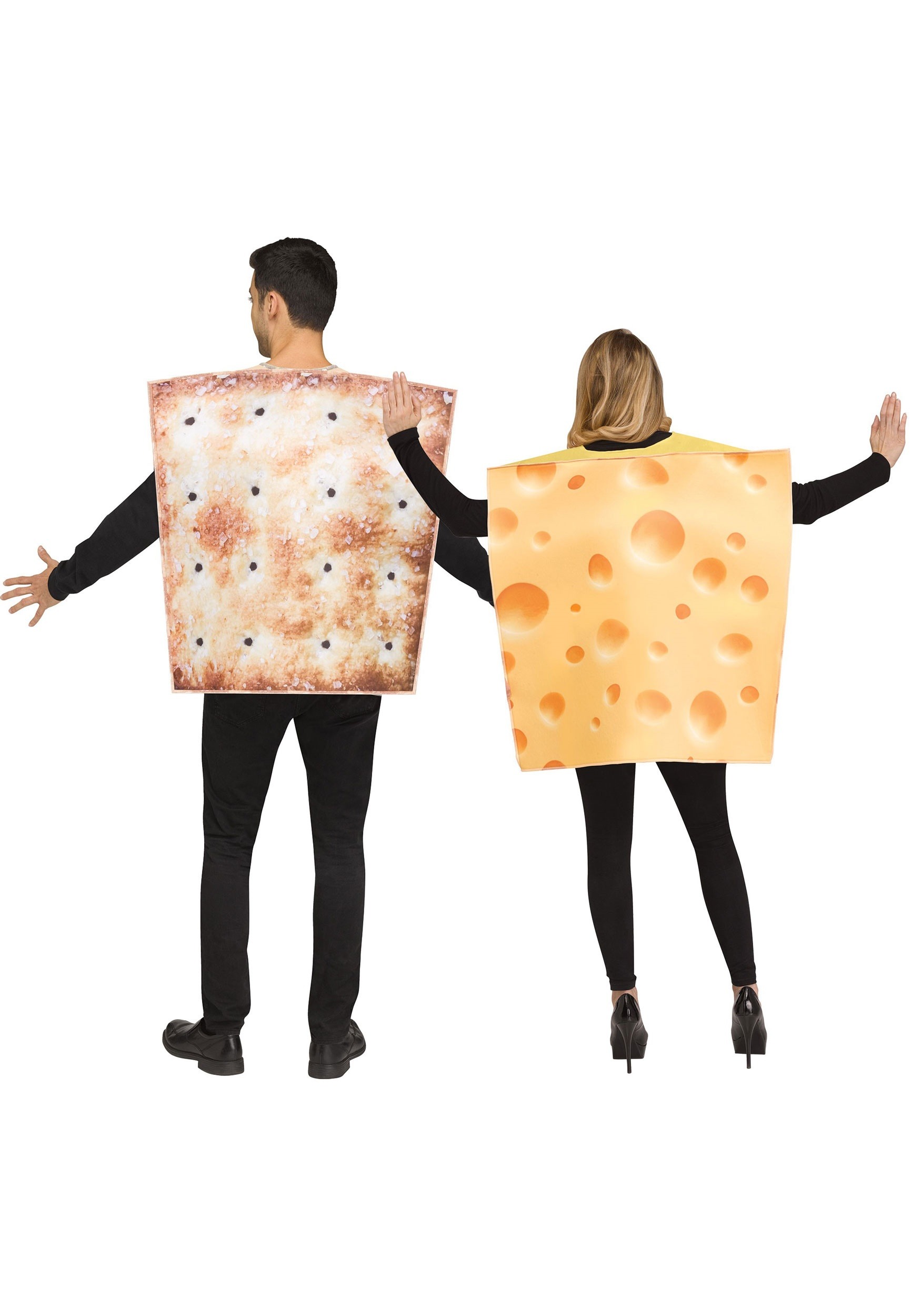This image features a male and a female model standing against a bright, white background. Both are dressed in black from head to toe; the man wears black dress shoes, pants, and a long-sleeved shirt, while the woman complements her black leggings and long-sleeved shirt with black patent leather high heels. Each is modeling a humorous, square-shaped costume that covers only their top torso; the man's costume resembles a saltine cracker, and the woman's a slice of Swiss cheese, complete with characteristic holes. With their backs facing the viewer and arms extended to the sides to fully display their costumes, the man, taller by about a head, sports short dark hair and a five o'clock shadow, while the woman, with shoulder-length blonde hair pulled to the front, has her elbows bent. The playful juxtaposition of the saltine cracker and Swiss cheese costumes creates a whimsical visual contrast.